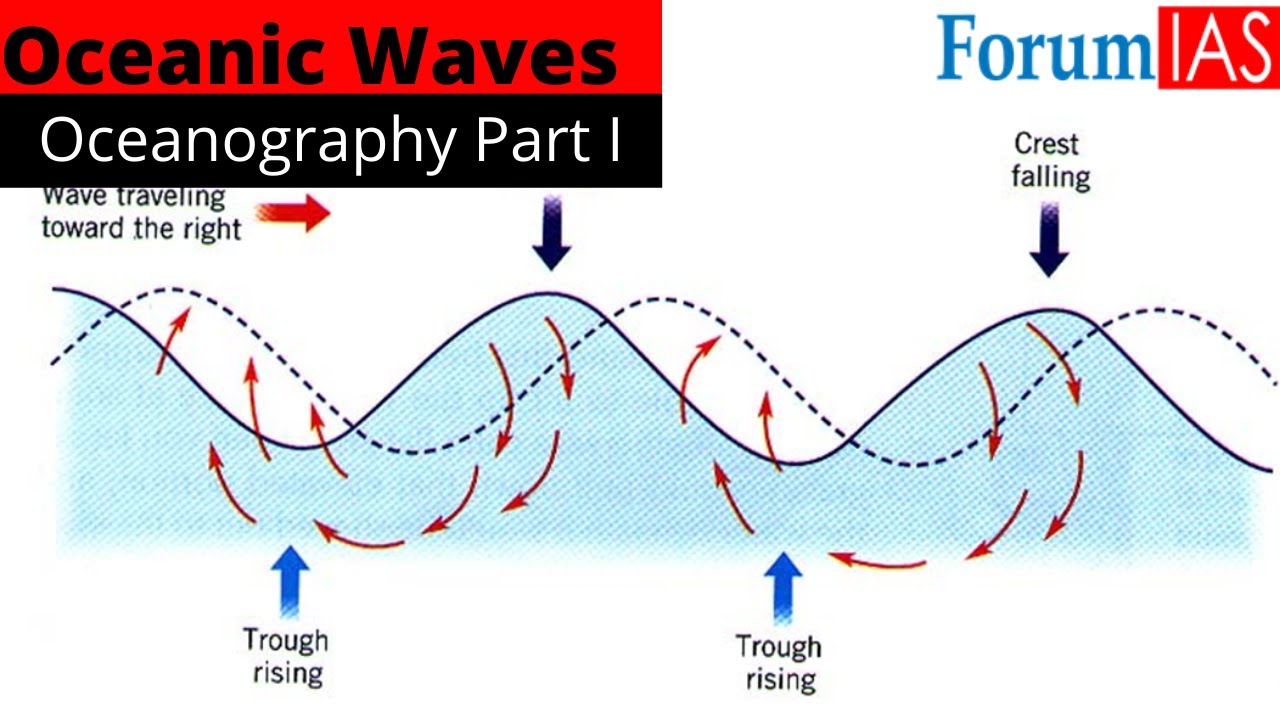The image is a scientific graphic focused on oceanic wave movements, primarily against a white background. At the top left corner, a box labeled "oceanic waves" is written in black with a red background, and directly below it, "oceanography part one" is written in white against a black background. In the top right corner, "forum" is written in blue text, whereas "IAS" is displayed in white text against a red background. 

The visual depicts two waves, one represented by a dotted line and the other by a solid blue-filled line. Red arrows circulate around the waves, indicating their motion and direction. There is a labeled red arrow just below the "oceanography part one" box, stating "wave traveling towards the right," with the arrow pointing right.

At the lowest part of the waves, blue arrows labeled "trough rising" point to the troughs, where the waves begin their upward movement. Additionally, darker blue arrows labeled "crest falling" indicate the crests' downward path. The overall graphic uses various colors to illustrate the dynamics of wave motion effectively.